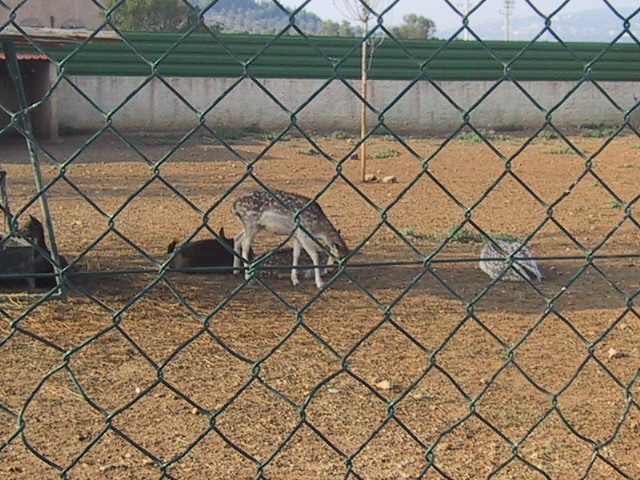This image, a rectangular outdoor photograph captured from behind a green chain-link fence, depicts an animal enclosure possibly located at a zoo or animal rescue center. The fenced area houses two deer-like animals, distinguishable by their brown coats adorned with white spots. One animal is seen grazing with its head lowered to the ground, while the other one lies down, facing away from the viewer, revealing its white-tailed hindquarters with a distinctive black stripe underneath. The ground of the enclosure is mostly barren soil, interspersed with a few straggling weeds and bits of hay. 

In the backdrop, a tall gray concrete wall with a dark green wooden finish at the top runs across the enclosure's far side. This wall appears to create a boundary, beyond which a forested mountain is visible, giving a hint of natural surroundings beyond the enclosure. A bare tree is also present within the enclosure, and a shaded area rests to the left of the green-topped barrier. Small patches of grass are noticeable towards the back right corner of the enclosure, adding slight greenery to the mostly sparse environment. The upper right corner of the image shows the outlines of a distant cityscape, under a bright and sunny sky.